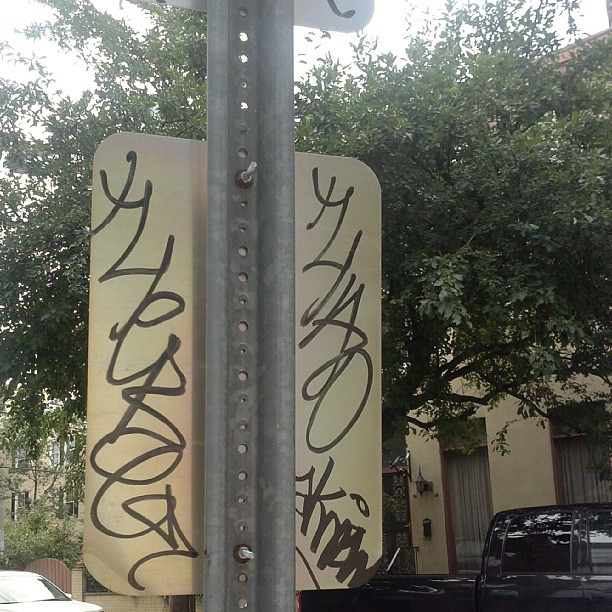The image depicts the back side of a street sign, attached to a gray metal pole secured with screws. The street sign is noticeably dirty, suggesting it hasn't been cleaned in a long time. The back of the sign is marred with illegible black graffiti, resembling sharpie scribbles. Centered in the photograph, the metal pole divides the sign, which extends out on either side. In the background, there is a light tan or cream-colored building, possibly a residence or apartment, with windows trimmed in brown and adorned with white curtains. A large tree stands behind the sign, adding a touch of nature to the urban setting. Below, a black pickup truck and a white car are parked along the curb, highlighting the typical daytime scene of a city street. The sun is shining, indicating that the photo was taken during the day.